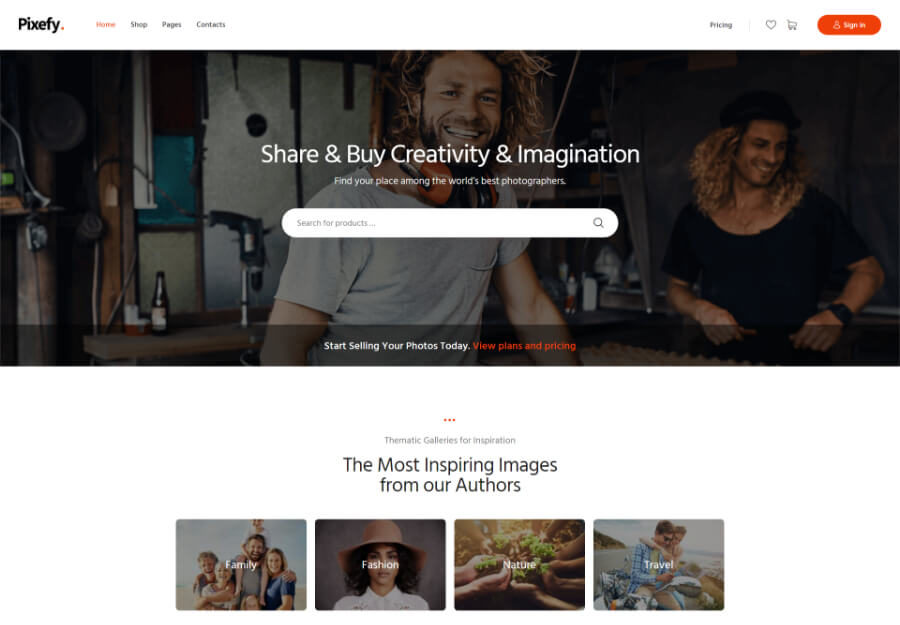The homepage of the Pixify website features a well-organized and visually engaging design. At the top-left corner sits the Pixify logo, composed simply of the word 'Pixify' followed by an orange period. Adjacent to the logo is a navigation menu with tabs labeled 'Home', 'Shop', 'Pages', and 'Contacts'. The 'Home' tab is highlighted in orange, indicating it is the currently selected page.

On the top-right side of the page, starting from the far right, there is an orange 'Sign In' button. To the left of this button, a series of icons and text follow: a shopping cart icon for accessing your cart, a heart icon for viewing your favorites, and the word 'Pricing'.

Dominating the upper half of the screen is a large, immersive image of two men smiling in what seems to be a bar. Superimposed at the center of this image are the words "Share and Buy Creativity and Imagination," followed by "Find Your Place Among the World's Best Photographers." Directly below these phrases is a search bar labeled "Search for Products." At the bottom of the image, centrally located, are the inviting words "Start Selling Your Photos Today," along with a notable link in orange, "View Plans and Pricing."

Scrolling down, the page introduces the 'Thematic Galleries for Inspiration' section. Here, the most inspiring images from Pixify's authors are presented in four clickable thumbnails:

1. A photograph of a family with the word 'Family' in the center.
2. An image of a woman with curly black hair, likely Hispanic or African American, wearing a large hat, labeled 'Fashion.'
3. A picture of a circle of hands holding green plants, centered with the word 'Nature.'
4. A snapshot of a couple snuggled on a scooter or motorcycle at the beach, captioned 'Travel.'

Each thumbnail image serves as a menu option that users can click to explore these themed photo categories. The backdrop of the entire layout is white, ensuring that the vibrant images and text stand out clearly.